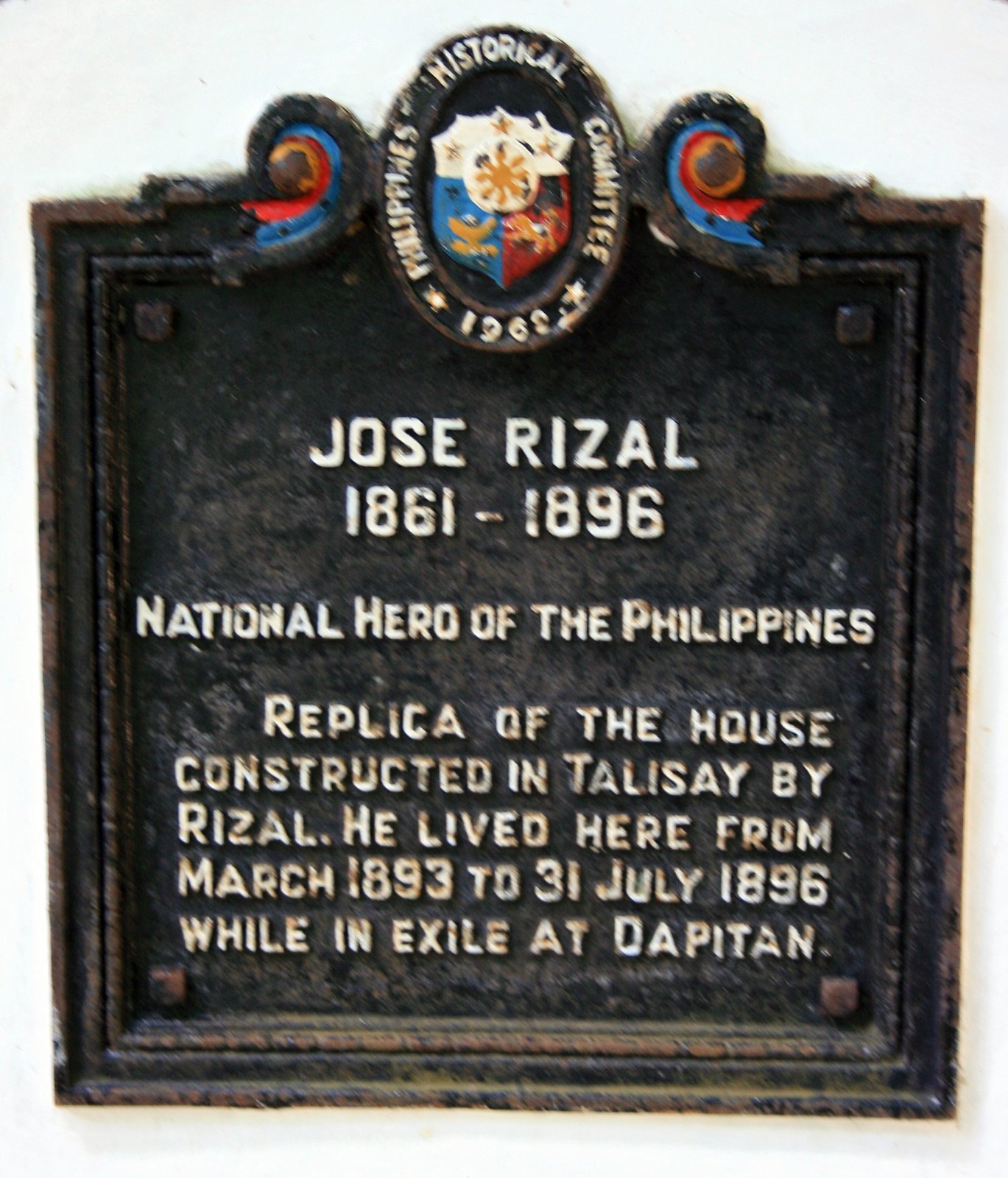The image is a black metal placard with a distinct square shape, except for the top where there is an oval. The placard has raised white-painted text that reads: "Jose Rizal 1861 to 1896. National Hero of the Philippines. Replica of the house constructed in Talisay by Rizal. He lived here from March 1893 to 31 July 1896 while in exile at Dapitan." Above the text, there is an oval logo that reads: "Historical Committee Philippines 1969," surrounding a crest shield. The shield is divided into three sections: a gold bird on a blue background on the bottom left, a winged lion on a red background on the bottom right, and a white section with yellow stars across the top. The background of the image is white, making the black placard and its details stand out clearly.